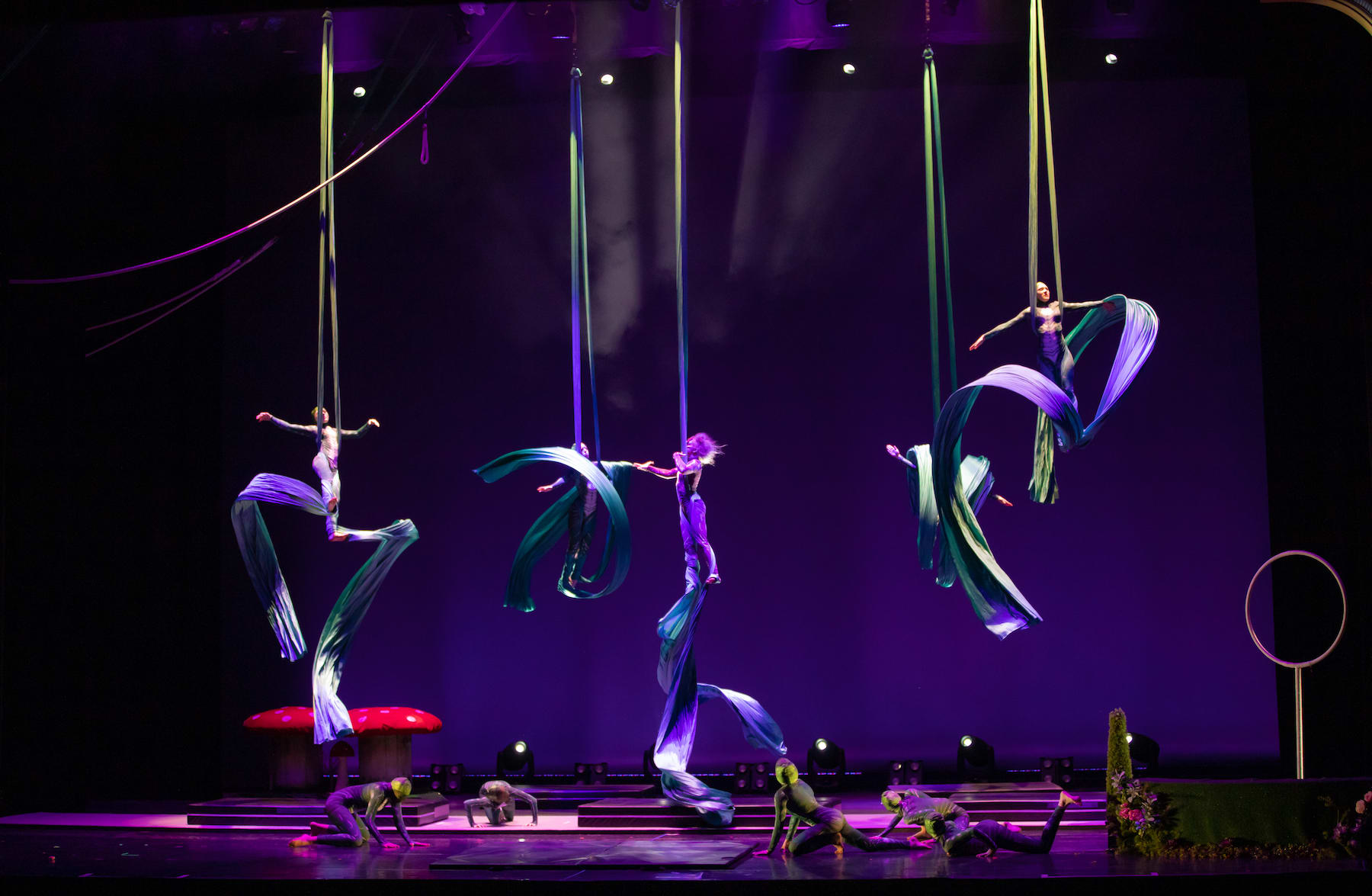This image captures a vibrant, theatrical performance set against a predominantly purple-lit stage. Suspended in midair, five aerial performers elegantly twirl and pose with the aid of oversized, colorful scarves that drape from the ceiling and cascade around their bodies and legs. Below them, on the stage floor, five individuals, seemingly dressed as green animals or frogs, engage in a performative dance, slithering and crawling towards a centrally located person dressed in purple. The scene is enriched with whimsical props, including two large mushrooms—each around four feet tall, with red and white tops and tan bases—adding to the fantastical atmosphere. The set also features a green platform adorned with flowers. Various lighting effects, including purple and green hues, illuminate the performers and backdrop, creating a magical, otherworldly ambiance.